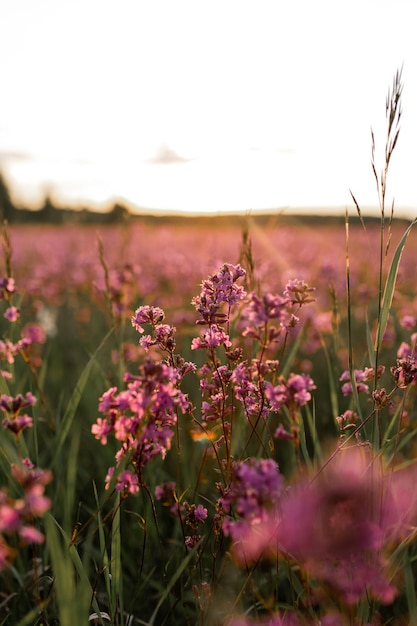The image is a close-up, photographic shot taken outdoors in a field during either the early morning or late evening. The central focus is a group of small, pinkish-purple flowers that appear almost like a bouquet, with some additional flowers to the left and right. These flowers have a cup-like shape and are illuminated by sunlight streaming overhead, creating a backlit effect that enhances their delicate hues. The background is a soft blur, suggesting a dimly visible expanse of greenery that could be a hillside or hilltop. Amid the green stalks and leaves, one particularly tall stalk extends toward the upper right-hand corner of the image. The sky above is white, dotted with a single dark cloud in the center and another faint dark cloud to the left. The image maintains a dreamy, soft-focus aesthetic, emphasizing the detailed, vibrant flowers in the foreground against a serene, out-of-focus background. The lower right-hand corner of the image is notably blurry, adding to the overall depth and atmosphere of the scene.